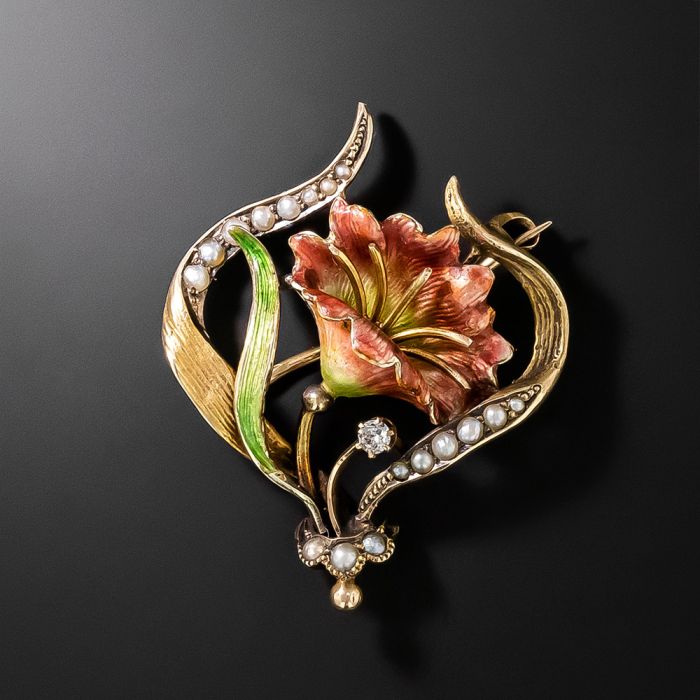The image showcases a refined piece of jewelry, specifically a brooch or pin, set against a black background. The design is centered around an elegant flower, reminiscent of a lily, predominantly adorned in muted red with touches of green and gold. The flower is complemented by lush, green leaves and a gold stem, further enriched with pearls and diamonds. The pearls, which are numerous and increase in size from the center towards the bottom of the piece, elegantly border the flower and embellish the leaves, adding a luxurious feel. At the base, a striking arrangement of three pearls leads to a prominent diamond, with an additional diamond accentuating the flower's petal-like structure. The overall heart-shape design is highlighted by the gold band framing the brooch, enhancing its opulence and making it a standout accessory likely intended for a lapel or coat.